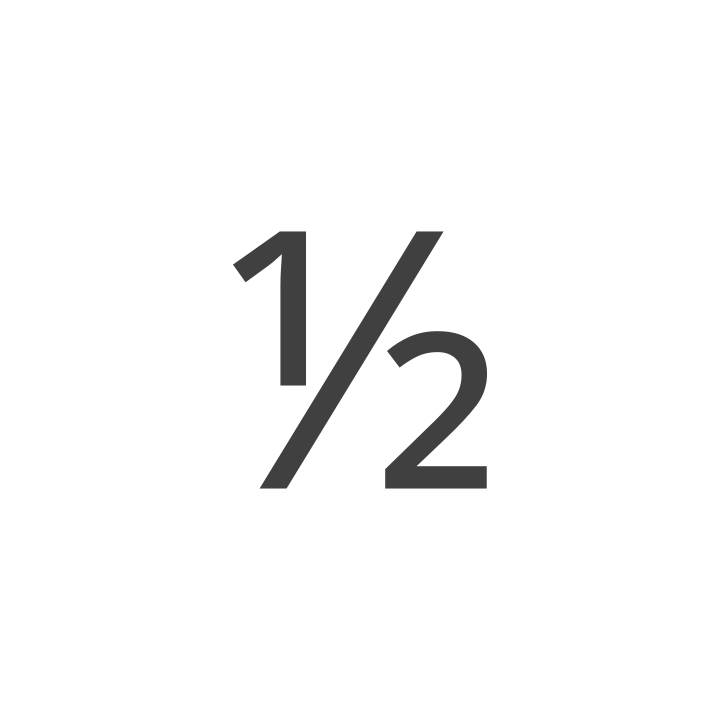The image illustrates a fraction "½" with a simple, clean design. The fraction is displayed in a very large, bold, dark gray font against a completely white background. The number "1" is positioned in the upper left, the diagonal slash is tilted slightly, and the number "2" is in the lower right, creating the staggered appearance typical of a fraction. The minimalistic and straightforward presentation emphasizes the numerical and fractional value of one half.